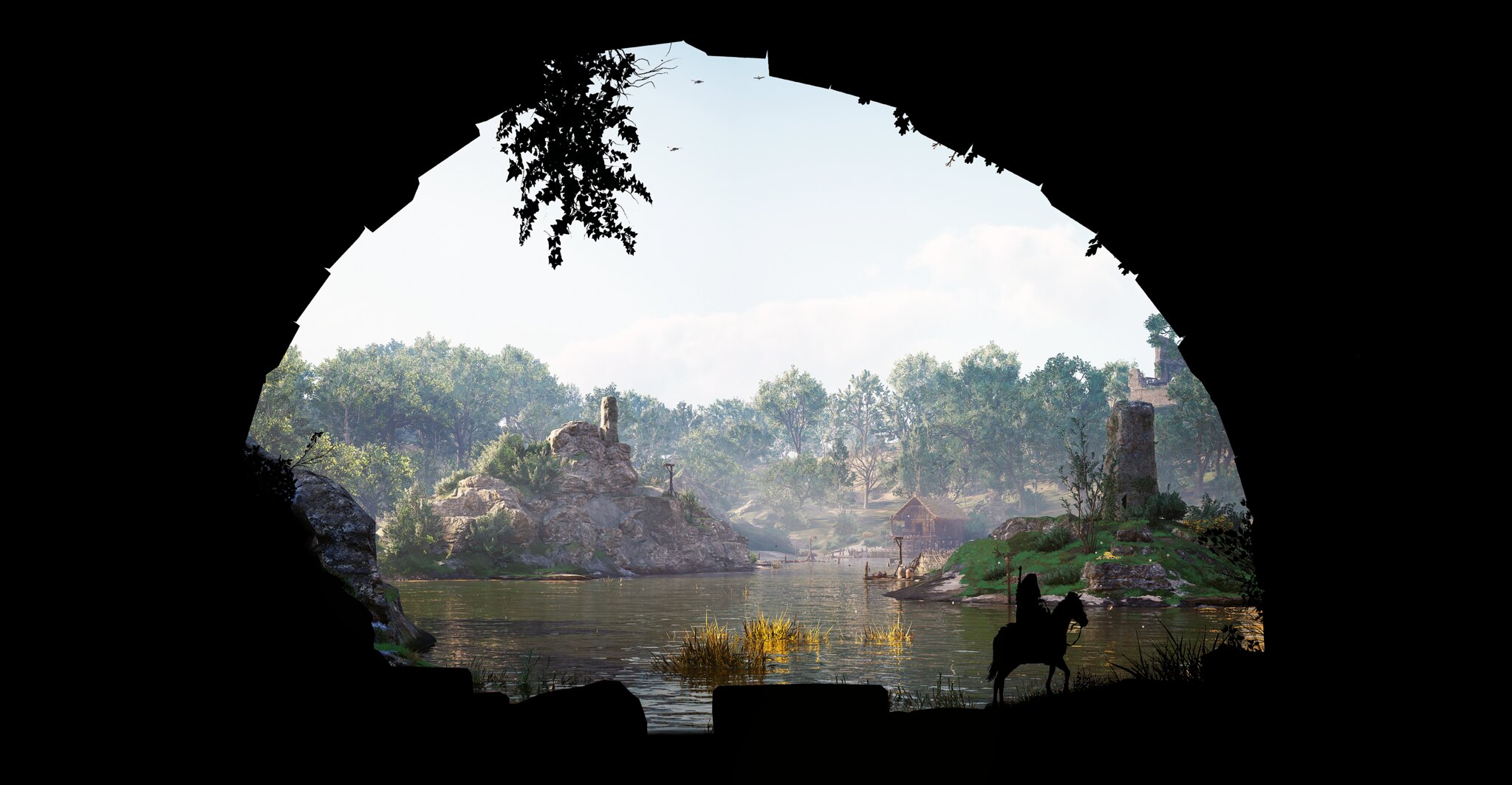A captivating image taken from within a shadowy cave, its rocky interior framing the scene. Jagged rock formations dominate the cave's floor and edges. Just above the cave's mouth, a small tree and scattered leaves hint at the world outside. Emerging from the cave's darkness, a horse and rider are highlighted against a tranquil lake. Across the water, a picturesque hill crowned with a quaint castle rises, flanked by trees. Another prominent hill features a similar castle, adding to the fairy-tale ambiance. In the background, a dense forest stretches towards a serene, light blue sky, completing this picturesque and enchanting landscape.